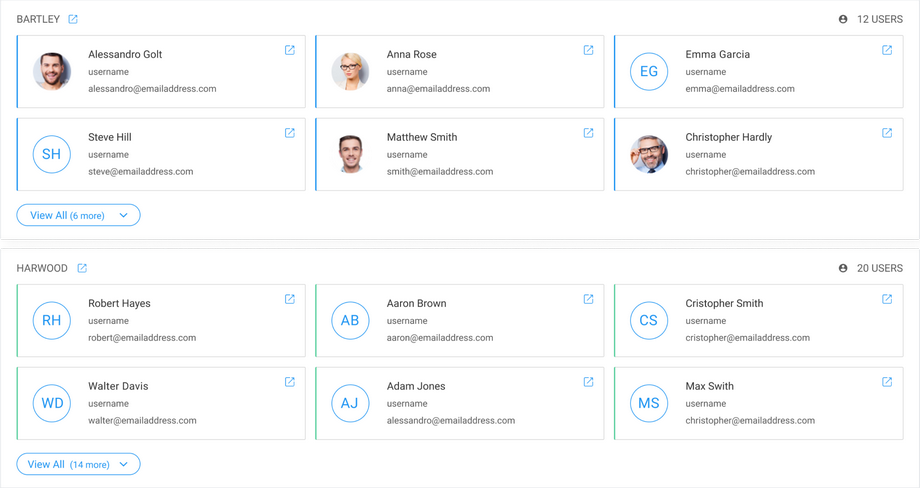In this detailed screenshot, displayed against a solid white background, we observe a grid of images and text boxes representing various users. In the upper left corner, there's an individual box containing the image of a young man with a beard, mustache, dark hair, and fair skin. His name, "Alessandro Golt," is displayed in black text alongside his username, "Alessandro," and his email address formatted as "alessandro@example.com." Directly to the right of Alessandro, there is a box featuring a female user with blonde hair and black glasses. Her name, "Anna Rose," is shown along with her username, "Anna," and her email address, "anna@example.com." 

Moving further to the right, there is a box without an image, instead showing the initials "EG" in blue text inside a circle, representing "Emma Garcia." Her username and email address ("emma@example.com") are also indicated below her name. In the upper right corner of the overall image, there's a label stating "12 users" in black text, highlighting the total number of users.

The upper left-hand corner of the box grid features the name "Bartley," written in black text. An additional note underneath indicates that there are six more users beyond the six currently visible in this grid.

Below this section, there is another rectangle outlined in light gray. In the upper left corner of this section, the name "Harwood" is displayed. Harwood manages a team of six members, all of whom are shown within this gray-outlined rectangle.